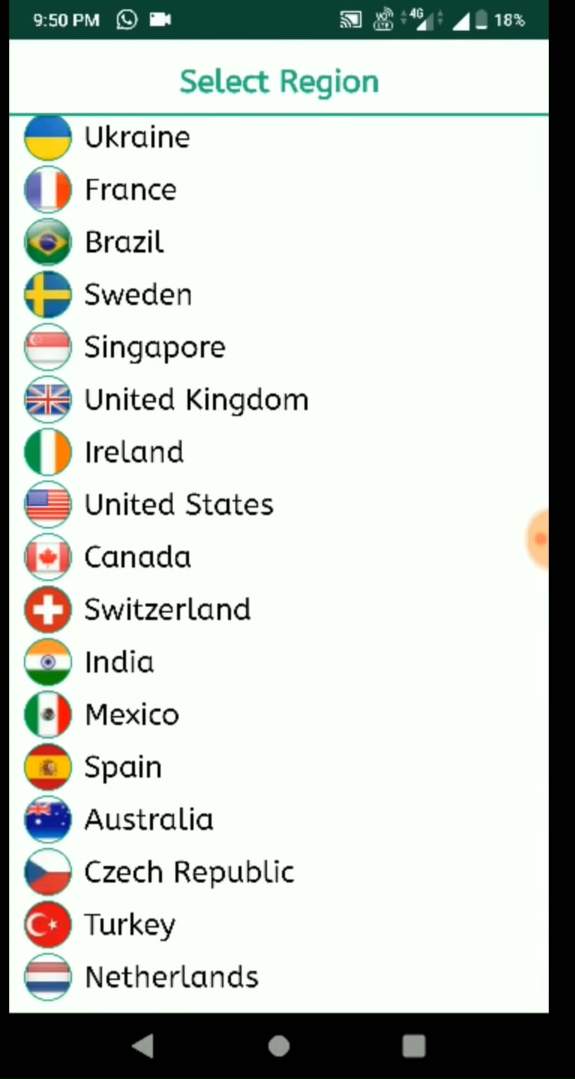The image displayed on a user's cell phone screen is a white vertical rectangle set against a black background. In the top left corner, the device time reads 9:50 p.m. To the right, icons for voicemail and video are visible, alongside indicators showing the phone has 18% battery life remaining and about half of the bars for 4G signal strength.

At the very top of the image, "Select Region" is written in teal-colored text, accompanied by a teal line that extends horizontally across the screen just below this heading. The main part of the screen features a vertical list of countries, each accompanied by its respective flag encased in a circular icon to the left of the country name. The countries listed are Ukraine, France, Brazil, Sweden, Singapore, United Kingdom, Ireland, United States, Canada, Switzerland, India, Mexico, Spain, Australia, Czech Republic, Turkey, and Netherlands.

At the bottom of the screen, there are three icons typically used for navigation: a back arrow, a home circle, and a square for recent apps.